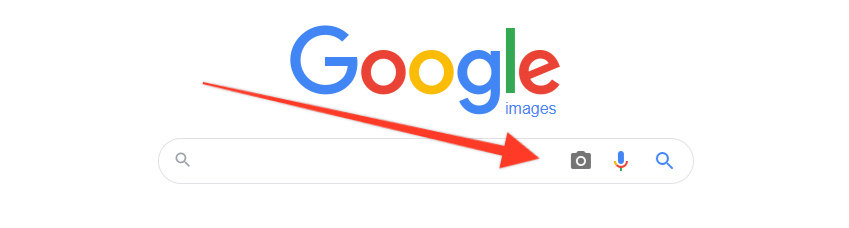The image depicts the Google homepage with the word "Google" prominently displayed in its iconic colors: blue, red, yellow, blue, red, and green. Beneath the letters 'L' and 'E' in "Google," the word "images" is written. The background is entirely white, with no additional pictures or text. A large red arrow points diagonally from the upper-left, at the same level as the 'G' in "Google," towards a small camera icon located in the search bar. The search bar also contains a gray magnifying glass icon on the left and a blue magnifying glass icon within the search box, immediately before the microphone icon. The overall simplicity and focus of the image emphasize the camera icon, suggesting the use of Google’s image search feature.